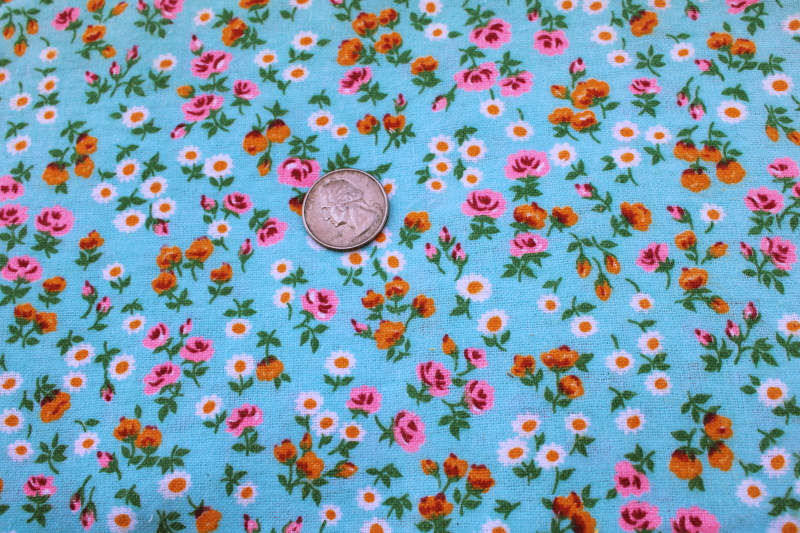The image is a photograph of a United States quarter, showcasing the head side with George Washington's profile. The quarter, appearing slightly worn, is positioned just left of center and slightly upwards from the middle of the frame. The background is a light, aqua blue fabric that might be a tablecloth or dress, covered in a detailed floral print. This print features tiny, feminine flowers: pink and red roses, white daisies with orange centers, and small gold flowers, with all flowers accompanied by green stems and leaves. Some flowers are in full bloom while others are in the bud stage, adding a dynamic touch to the pattern.